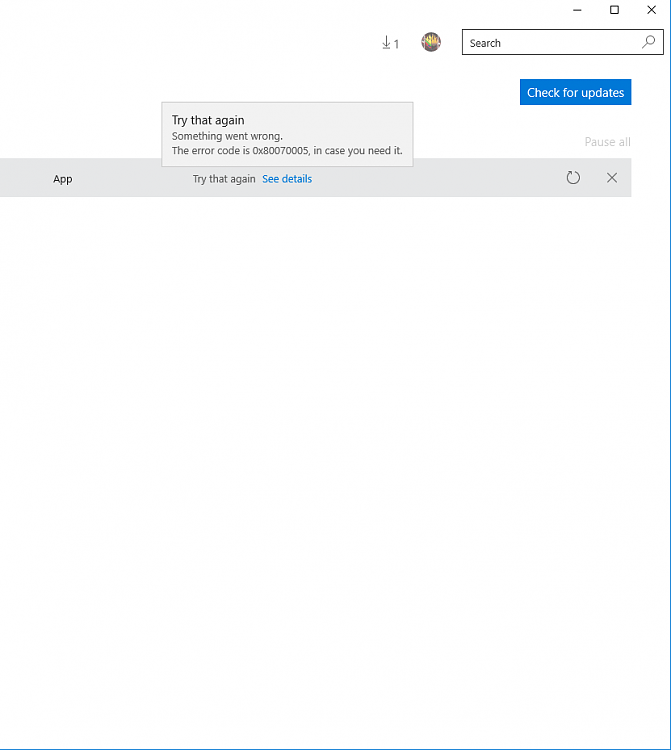The image captures a screenshot of a Windows error page. Dominating the screenshot is an error box overlaid on a typical Windows settings interface. In the top-right corner, the window features the customary minimize, maximize, and close buttons. Below these, the search bar is equipped with a magnifying glass icon on the left, followed by a profile picture, and to the left of this is a download icon indicating one active download.

Situated beneath the search bar is a prominent blue button labeled "Check for updates," with a gray "Pause all" option directly below it. Further down, a thick gray line spans horizontally, containing the word "App." Following to the right of "App," the text reads "Try that again," "See details" in blue, "Reload," and an "X" to close.

Central to the image, an error message box overlaps the gray line and a portion of the white background space. This gray error box prominently displays "Try that again" in bold text, followed by "Something went wrong." It lists the error code as "0x80070005 in case you need it."

The remaining portion of the image is largely composed of empty white space, with a blue outline encircling the perimeter of the screenshot.